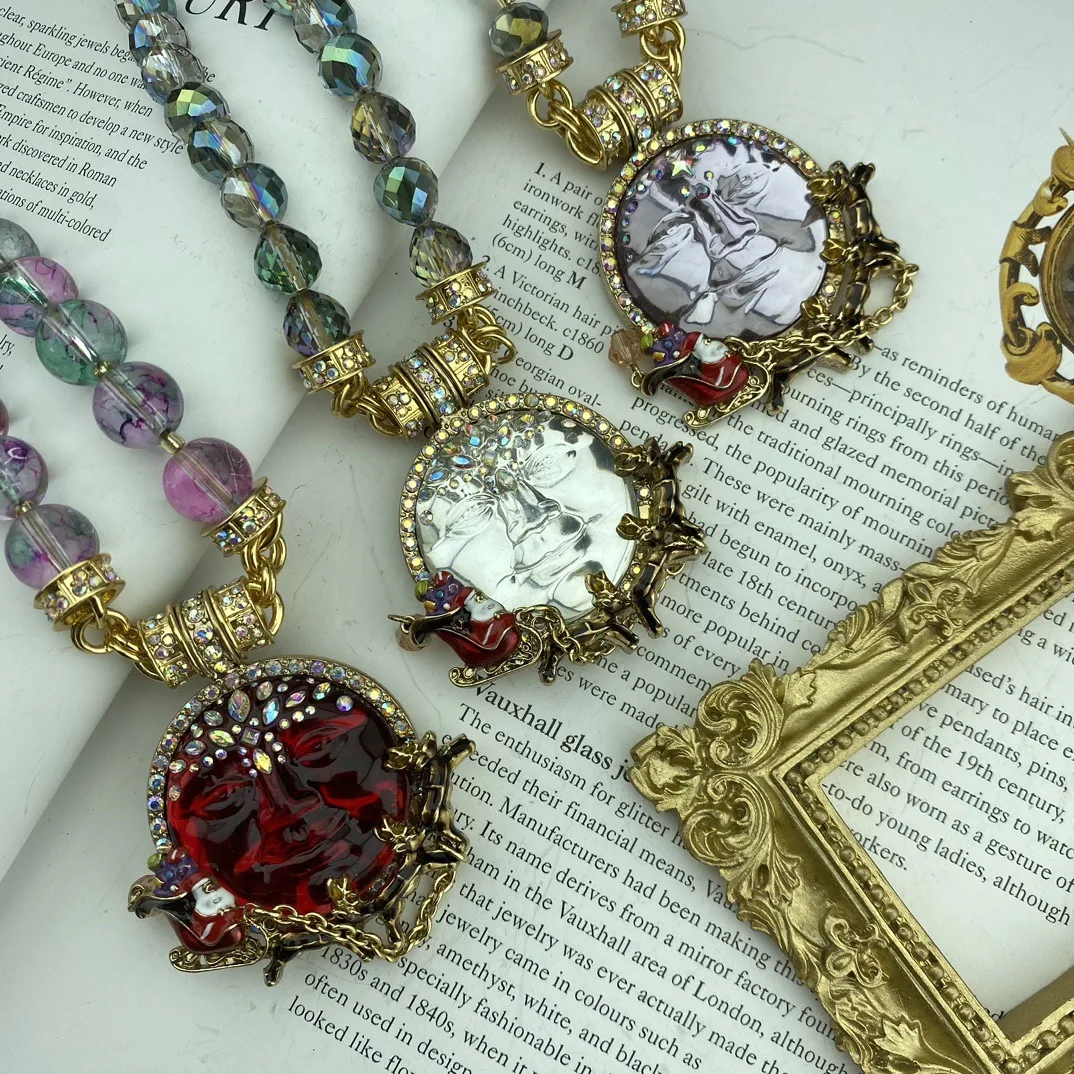The image depicts three elaborately adorned necklaces resting diagonally from the top left to the bottom right on an open book with black text on white pages. Each necklace features a circular pendant, each with a distinct face, adorned with various jewels. The first necklace, the farthest on the right, has a gemstone-encrusted red face and a chain made of purple and green beads linked by a gold clasp with decorative rings. The pendant is further embellished with a depiction of Santa Claus in a sleigh, pulled by reindeer, wrapping around the base. The second necklace, to the right of the first, features silver, clear, and blue beads with a similar gold clasp and pendant design—a jeweled silver face with additional ornamentation on the forehead. The third necklace has a less-visible chain but shows a silver-colored pendant with intricate decorations and likely similar thematic elements. Additionally, on the right side of the image, there is a partially visible gold frame, hinting at an ornate picture frame angled toward the bottom. The composition is rich with metallic hues and intricate details, giving an overall impression of ornate, vintage jewelry craftsmanship.